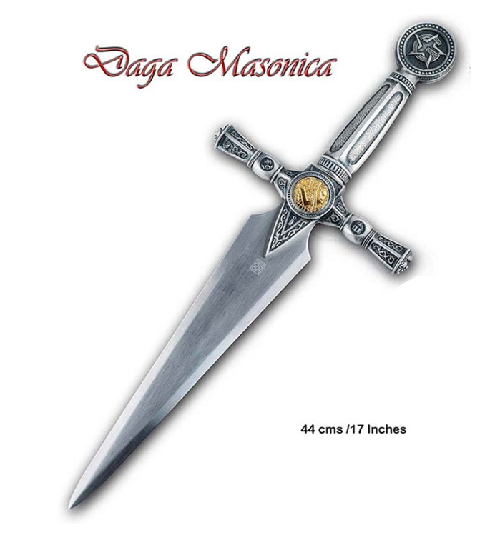The image depicts a medieval-style dagger positioned on a wide, white background. The silver dagger features a sharp, double-edged blade that tapers to a fine point, with a lighter silver hue along the edges indicating its sharpness. The handle is intricately designed and includes a vertical crossguard with flared ends that prevent the hand from slipping onto the blade; these ends have detailed etchings in black and silver. 

At the top of the handle, where it meets the blade, is a round piece adorned with a gold-toned gem resembling a clear yellow jewel. The very end of the handle, where the pommel is located, includes a round design with a star motif, also gold-hued, possibly signifying a decorative jewel. Alongside the ornate handle, there are slits and grooves to improve grip.

The dagger's detail is further enhanced by red cursive text reading "Daga Masonica" located in the upper left of the image, and the dimensions "44 CMS / 17 inches" appearing in the bottom right corner, indicating the full length of the dagger. The overall craftsmanship and decorative elements suggest an antique or ceremonial use.